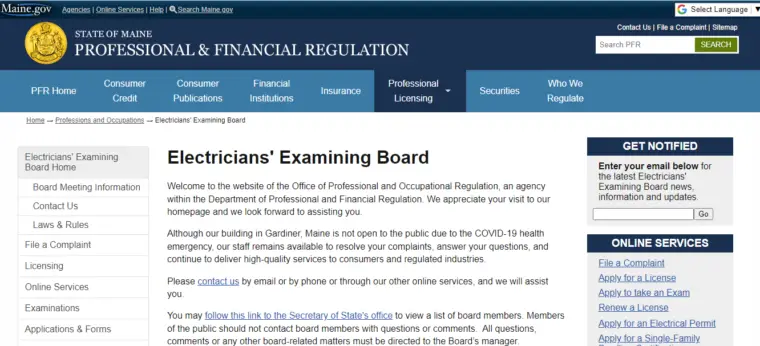Here's a cleaned-up and detailed caption for the image described:

"The web page from Maine.gov is designed with a comprehensive layout. On the left-hand side, under the 'Maine.gov' header, there are links for 'Agencies' (underlined), 'Online Services,' and 'Help,' all presented as clickable buttons. A magnifying glass icon accompanies the text 'Search Maine.gov.' Following this, the seal of Maine is displayed within a gold circle, and underneath it, bold white text reads 'State of Maine.' Below that, another segment states 'Professional and Financial Regulation' in all caps. 

A light blue rectangle appears further down, contrasting with the dark blue rectangle on the right that reads 'Search PFR' and contains a small green button labeled 'SEARCH' in all caps. Above this green button are links for 'Contact Us,' 'File a Complaint,' and 'Sitemap,' all aligned in a light gray rectangle featuring a Google logo, with a dropdown option labeled 'Select Language' indicated by a black arrow.

In the light blue section, a navigation menu lists 'PFR Home,' 'Customer Credit,' 'Consumer Credit,' 'Consumer Publications,' 'Financial Institutions,' 'Insurance,' and 'Professional Licensing.' 'Professional Licensing' is highlighted in dark blue to show selection, with a down arrow suggesting additional options. 'Securities' and 'Who We Regulate' follow in the list. 

To the left within a gray rectangle against a white background, a secondary menu lists 'Electricians' Examining Board Home,' which is currently selected, followed by 'Board Meeting Information,' 'Contact Us,' 'Laws and Rules,' 'File a Complaint,' 'Licensing,' 'Online Services,' 'Examinations,' and 'Applications and Forms.'

Above this secondary menu, outside the gray rectangle, breadcrumb navigation is displayed: 'Home' (underlined) leading to 'Professions and Documentations,' and finally 'Electricians' Examining Board,' which is bolded in black to indicate the current page."